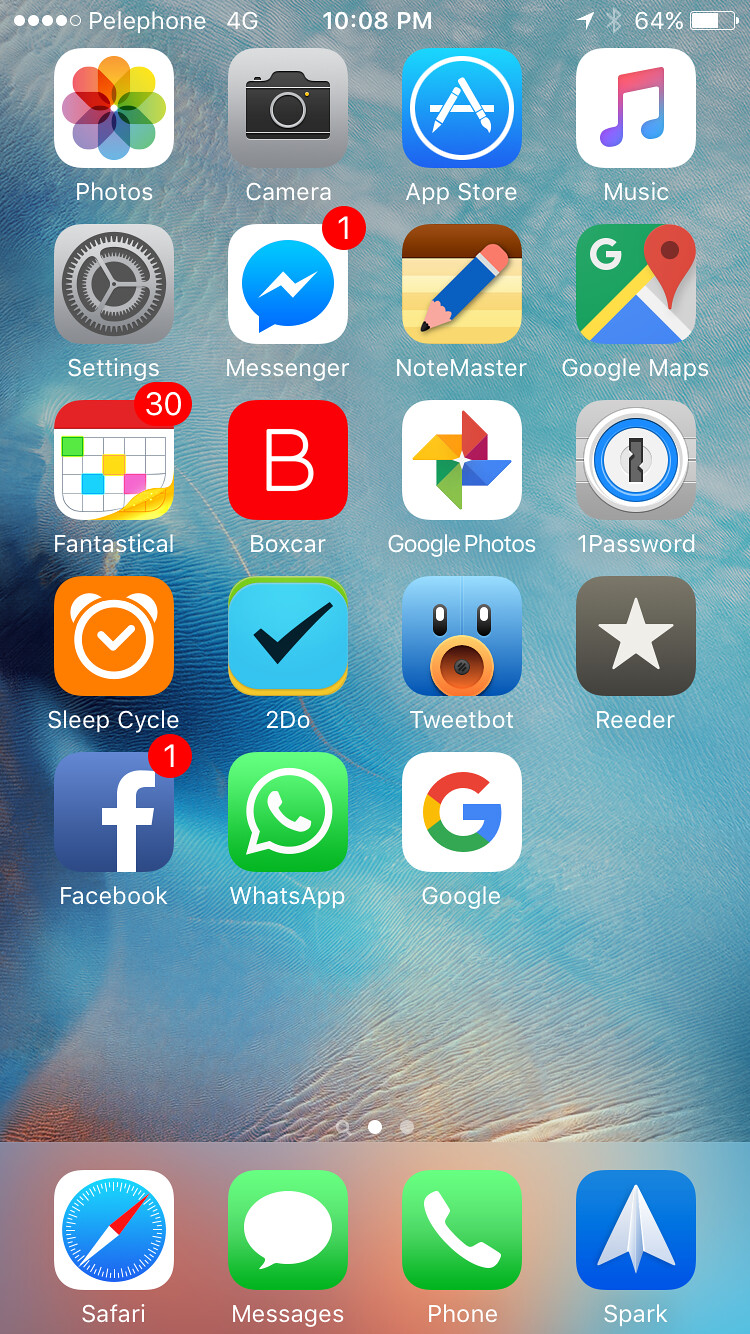Screenshot of an iPhone Displaying the App Menu

The image is a detailed screenshot of an iPhone's app menu screen. The wireless provider at the top left corner shows "Pelephone 4G", and the current time is 10:08 PM. The status bar also displays navigation and Bluetooth icons, along with a battery life indicator at 64%.

The app icons are neatly organized in a grid from left to right and top to bottom, starting with:
1. Photos
2. Camera
3. App Store
4. Music
5. Settings
6. Messenger
7. Notemaster
8. Google Maps
9. Fantastical
10. Boxcar
11. Google Photos
12. 1Password
13. Sleep Cycle
14. To-Do
15. Tweetbot
16. Reader
17. Facebook
18. WhatsApp
19. Google

This is one of the two available app pages.

At the bottom dock, the icons are:
1. Safari
2. Messages
3. Phone
4. Spark

The iPhone’s background is a captivating top-down photograph of the ocean captured during sunrise or sunset. The lower half of the water has an enchanting orange hue, likely reflecting the sunlight. Additionally, a boat is visible traversing the water, creating noticeable waves and adding a dynamic element to the serene backdrop.